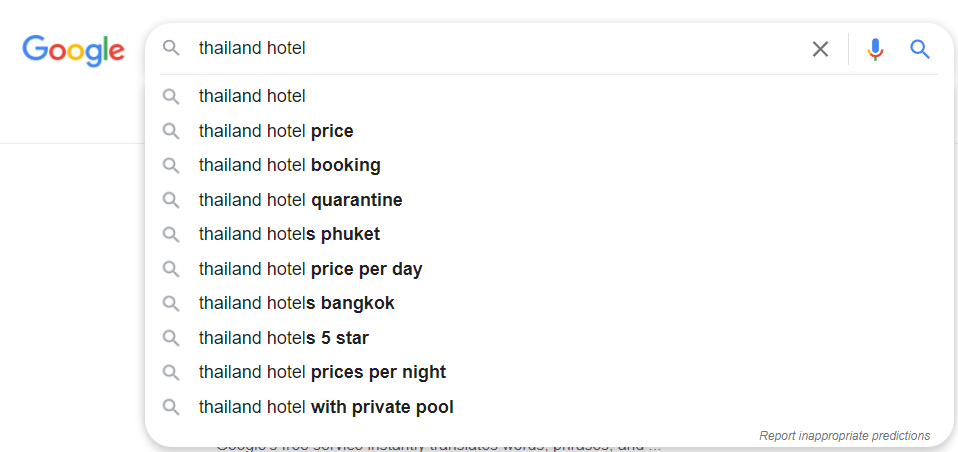The image portrays a screenshot of a Google search query where the user has typed "Thailand hotel." Below the search bar, a dropdown menu displays a list of suggested search queries that reflect common searches made by other users. The suggestions include: "Thailand hotel price," "Thailand hotel booking," "Thailand hotel quarantine," "Thailand hotels Phuket," "Thailand hotel price per day," "Thailand hotels Bangkok," "Thailand hotels five-star," "Thailand hotel prices per night," and "Thailand hotel with private pool." These auto-suggestions are designed to help users quickly refine their search without having to type out additional terms manually. The options provide a convenient way to navigate directly to specific information, ensuring a more efficient search experience.